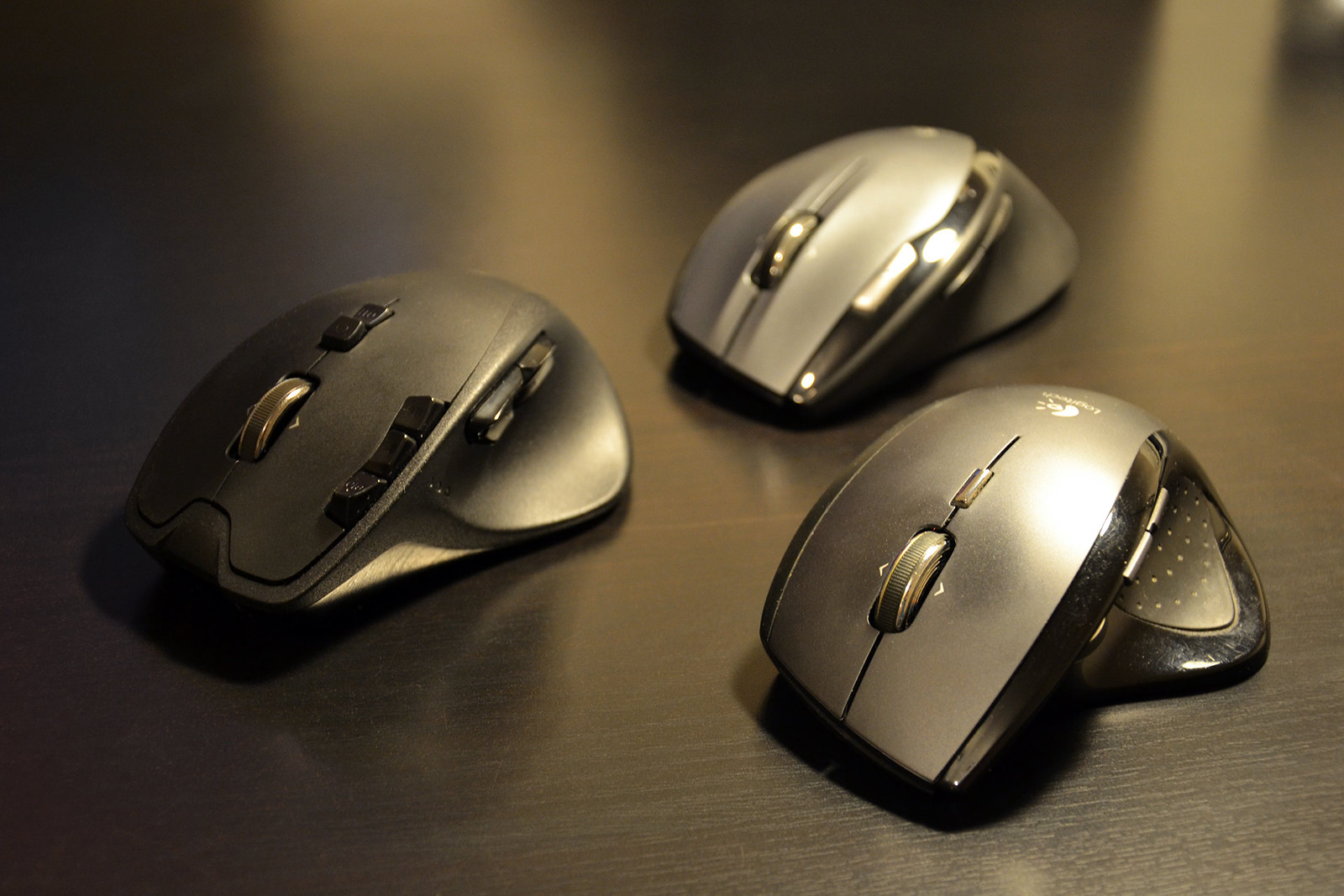In this image, we have a sleek, glossy brown table with darker shades and shadows. On the table, there are three wireless computer mice. Each mouse features a rolling trackball at the top and a thumb rest. Two of the mice, positioned on the left, are identical in size and shape but differ slightly in color; one has a black tab on the side while the other has a silver tab. The third mouse, placed on the right, stands out with a black rubber grip adorned with dots on the side. The mouse at the center, slightly elevated above the others, has additional buttons below and to the side of the trackball, suggesting it’s designed for users with different needs. All three mice have a silver and black design, possibly indicating they are from the Logitech brand. The image is illuminated from the top, causing some reflections on the glossy table surface.